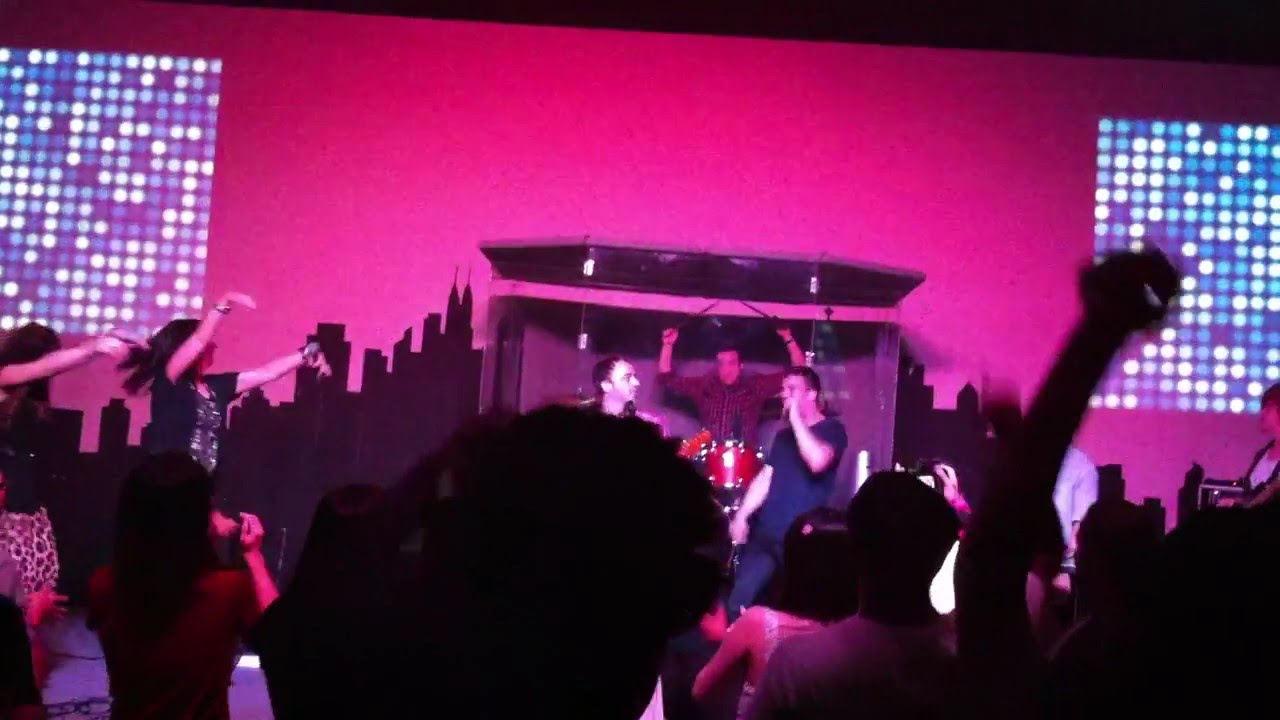This horizontal rectangular image captures a lively performance inside a nightclub. The scene is bathed in pink and purple hues, reflecting a vibrant and energetic atmosphere. In the background, a wall with a pinkish color dominates, adorned with two square decorations made up of smaller blue squares on either side. The backdrop also features the silhouette of a city skyline.

On stage, three performers are clearly visible. One, positioned behind a drum set, has both hands in the air, holding drumsticks, poised to strike. Another performer, a man in a dark t-shirt, holds a microphone, engaging with the audience. A third individual, partially obscured, appears to be another vocalist or DJ.

In the foreground, the animated audience is silhouetted, their arms raised, some dancing and others snapping photos with their cameras or cell phones. The scene is dynamic, with heads bobbing in rhythm to the music, creating a sense of communal enjoyment. Despite the poor image quality—blurry and slightly pixelated, likely from a video screenshot—the infectious energy of the live performance is palpable.